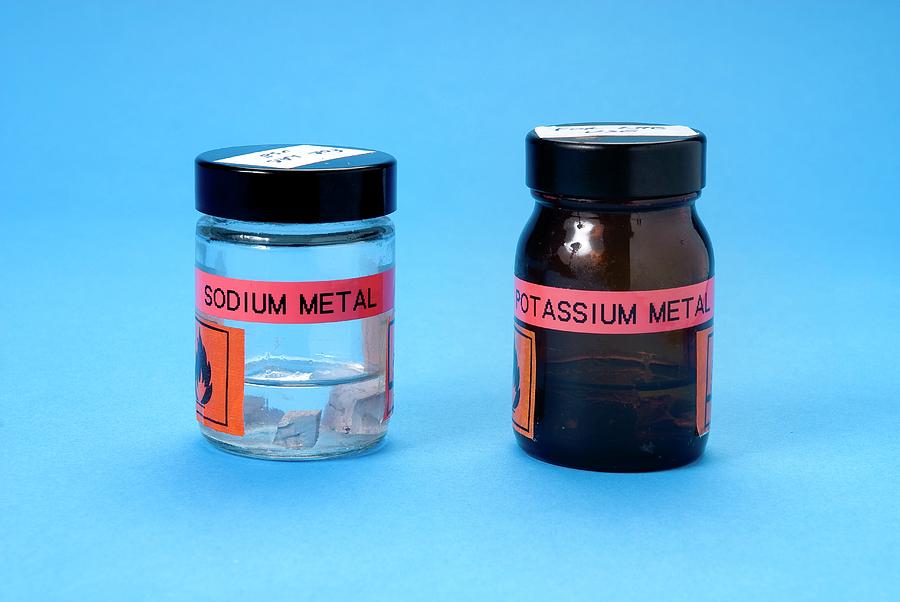The image features two short, wide glass jars set against a light blue background, possibly a tabletop or paper. The jar on the left is clear with a black lid, featuring a red label that reads "Sodium Metal" in black uppercase letters. Below this label, there is an orange flammable sticker displaying a black flame symbol. Inside this jar, which is about a quarter filled with clear liquid, are blocks of sodium metal in varying sizes, appearing gray and metallic. The right jar is a darker amber or brown-tinted glass, also with a black lid. This jar has a red label reading "Potassium Metal" in large black letters, and similarly to the left jar, it has an orange flammable sticker below the label. The contents of the right jar, though partially obscured by the tinted glass, also include liquid and possibly solid chunks of potassium metal. Both jars have a piece of masking tape on their lids with illegible writing.